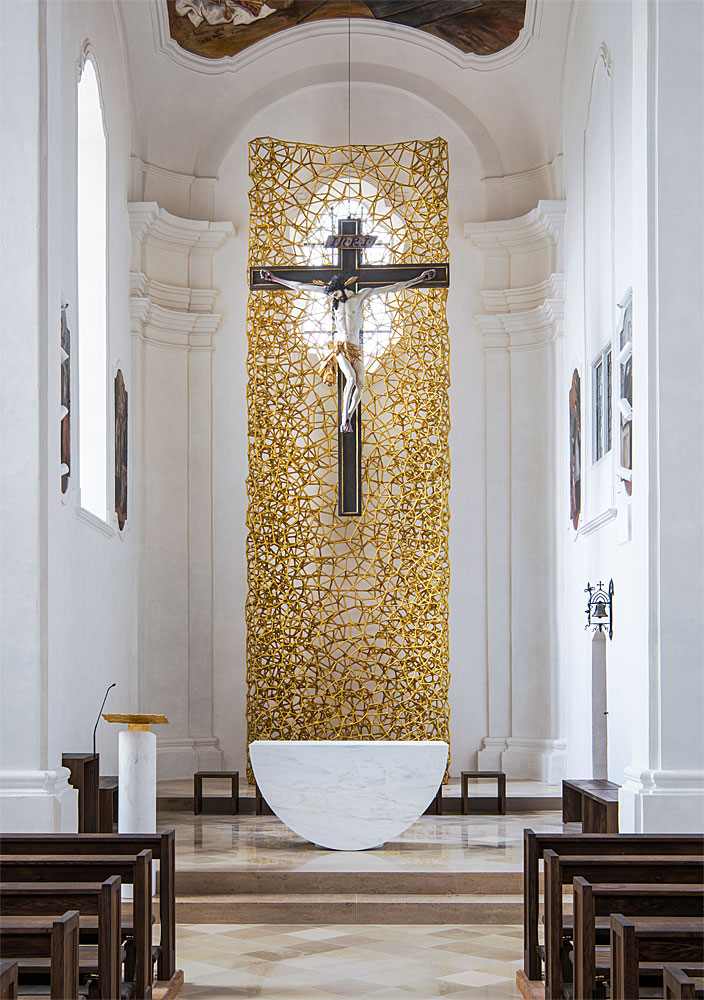The photo captures the interior of a modestly sized church, focusing on the front area with about four rows of brown wooden pews visible. The church features white-painted walls and a high ceiling, creating a spacious and airy atmosphere. Dominating the center of the image is the altar, backed by an intricate tall gold net-like structure. Attached to this structure is a sizable rectangular brown cross, bearing an inscription of "INRI" and with Christ hanging on it. Behind the cross, there is a faint light that adds a spiritual illumination to the scene. Additionally, a pulpit with a half-circle, possibly marble, white base, is positioned near the gold structure. The floor of the church showcases square marble tiles in shades of gold, brown, and white, contributing to the elegant and serene ambiance of this sacred space.